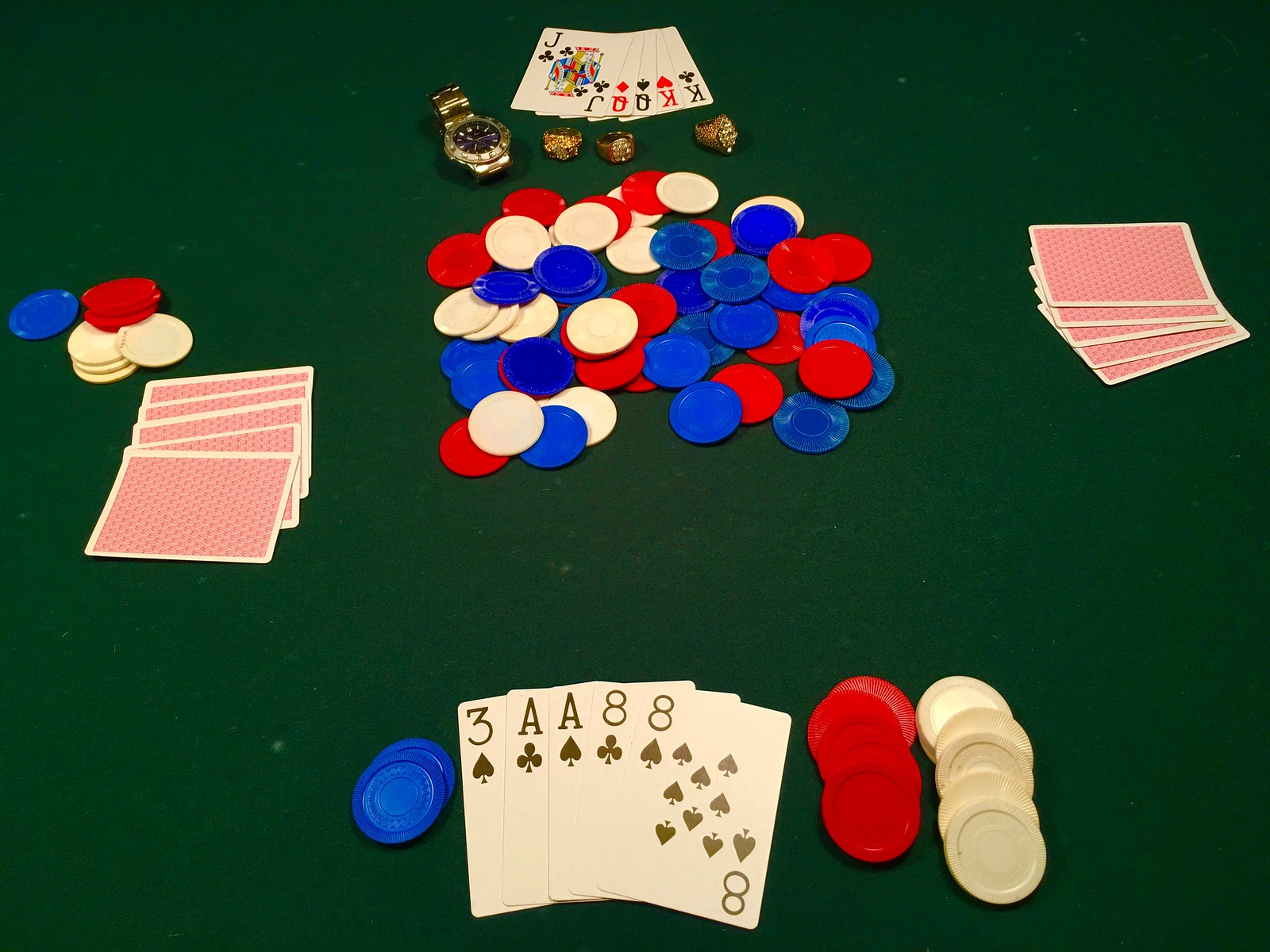The image showcases four distinct poker hands positioned against a green felt table. The layout is as follows:

- **Top Hand:** This hand is displayed face up, revealing a combination of a Jack of Clubs, 8 of Diamonds, 8 of Spades, King of Hearts, and King of Clubs. Surrounding this hand is an array of luxurious accessories, including a golden watch and three golden rings, each adorned with what appear to be diamonds.

- **Bottom Hand:** Also face up, this hand consists of five black cards: a 3 of Spades, Ace of Clubs, Ace of Spades, 8 of Clubs, and 8 of Spades. To the left of this hand are a couple of blue poker chips, while to the right is a stack of red and white chips.

- **Left Hand:** Positioned face down, this hand displays a red, grid-like pattern with a white border on the back of the cards. Accompanying this hand on its left side is a small stack of poker chips in white, red, and blue.

- **Right Hand:** Similarly face down, this hand also shows the red, grid-like pattern on the back. It is notably devoid of any poker chips around it.

In the center of the table, a mix of blue, white, and red poker chips are scattered, adding to the vibrant and competitive atmosphere of the scene.